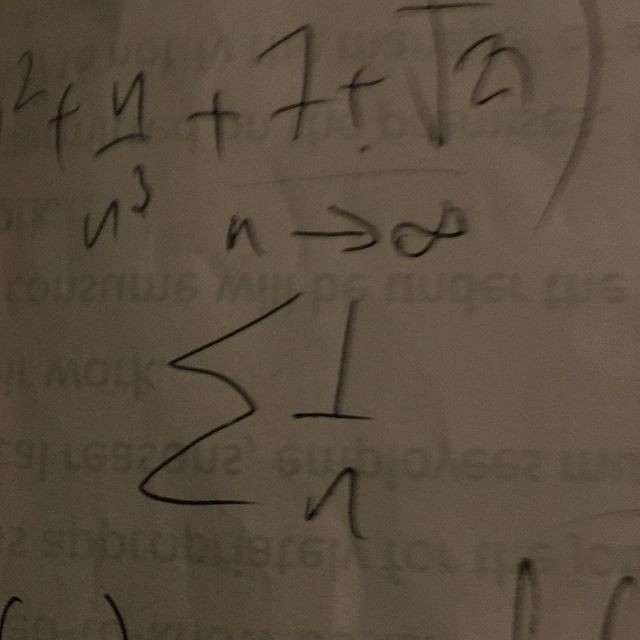This photograph captures a piece of paper covered in handwritten mathematical equations. The paper itself appears worn, with faint, indistinct text from the opposite side bleeding through, suggesting it is written in a non-English language characterized by longer words and unique punctuation. The math equation is rendered either in pencil or a black pencil crayon and contains a series of complex symbols, including an arrow pointing to the right and an infinity symbol prominently placed in the center. Brackets and plus signs are also visible at the top of the equation. The overall image suffers from poor lighting, casting deep shadows that obscure much of the detail. The white paper appears dim and shadowy, contrasting starkly with the dark handwriting. This creates a somber, almost murky visual experience.